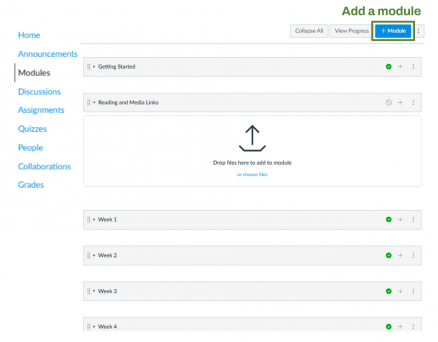A screenshot captures a minimalistic, behind-the-scenes view of a website, predominantly white in color. At the very top, against a white background, is a button labeled "Add a Module" situated to the far right. This button presents three options, with the third option highlighted in blue with white lettering, although the specific choice is indiscernible.

On the far left, a blue sidebar lists various navigation options: Home, Announcements, Modules (currently selected and displayed in black), Discussions, Assignments, Quizzes, People, Collaborations, and Grades.

The main screen is divided into sections, beginning with "Getting Started" at the top, followed by another section with blurred text. There is also a visible download icon. Below these headers are four more indistinct sections, likely labeled "Week 1," "Week 2," "Week 3," and "Week 4," each featuring a green dot on their right side.